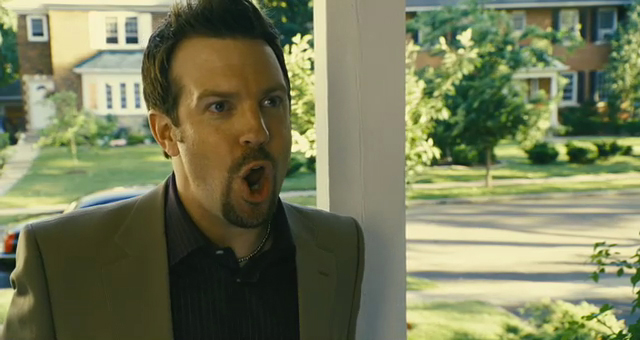This image captures Jason Sudeikis in what appears to be a scene from a movie, suggested by the wide shot framing. He is standing on a porch, dressed in a brown suit jacket with a distinctive dark brown, striped undershirt and a golden necklace. His facial hair is thin and stubbly, forming a goatee around his lips and chin, while his hair is slicked up at the front and down on the sides. Sudeikis’s mouth is open in a pronounced “O” shape, indicating he could be in the middle of exclaiming something. The background reveals a suburban setting with a white porch beam beside him, some neatly manicured lawns, and a parked blue car visible through the red taillight, with an assortment of two-story brick houses—one red and one orange with black shutters—framing the neighborhood scene behind him.